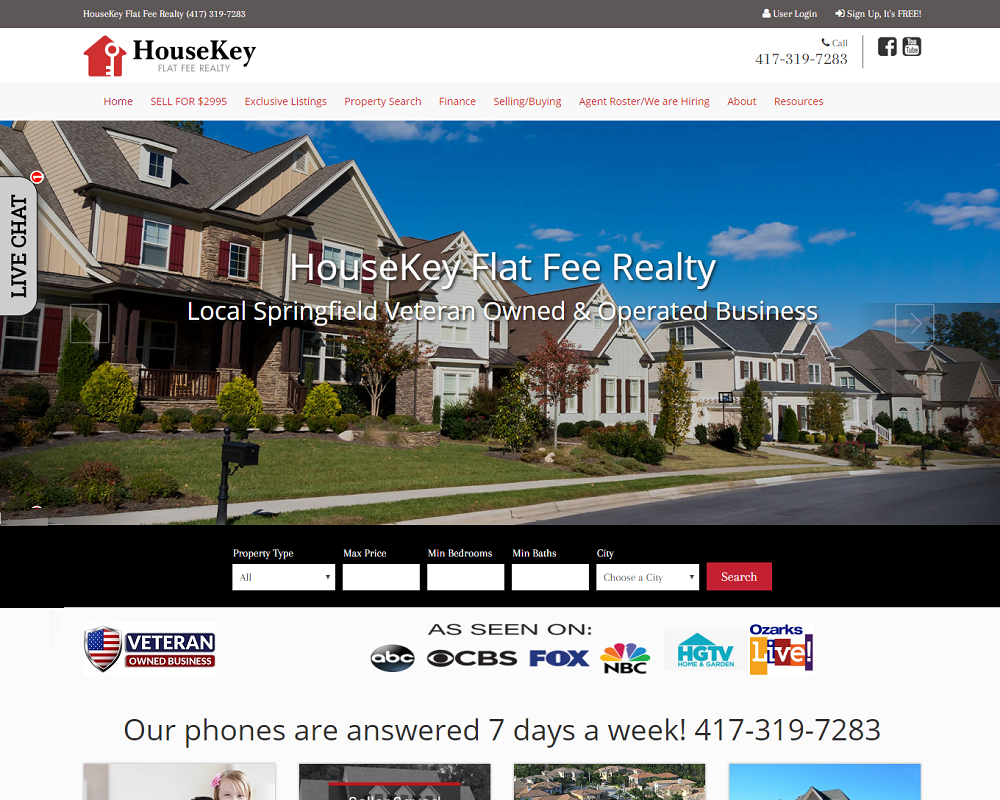Screenshot of a website titled "House Key" featuring a vibrant red house logo. The header below reads "House Key Flat Fee Realty." Prominently displayed is an image of a large, tan residential house situated within a neatly-kept neighborhood. The lawn is lush and green, and a paved street runs in front of the house. The sky above is a serene blue, dotted with white clouds, providing a picturesque backdrop.

At the bottom of the image are six boxes, five white and one red. The bottom left white box contains text stating "Veteran." Adjacent to it, text reads "As seen on ABC, CBS, Fox, NBC, HGTV, and something live." It also assures viewers that their phones are answered seven days a week, and provides a contact number: (417) 319-7283.

The text on the website is presented in black font, with a gray border at the top. Four separate photos are partially visible at the bottom, showing only their upper sections. Additionally, a Facebook icon is located at the top, alongside the phone number: (417) 319-7283.